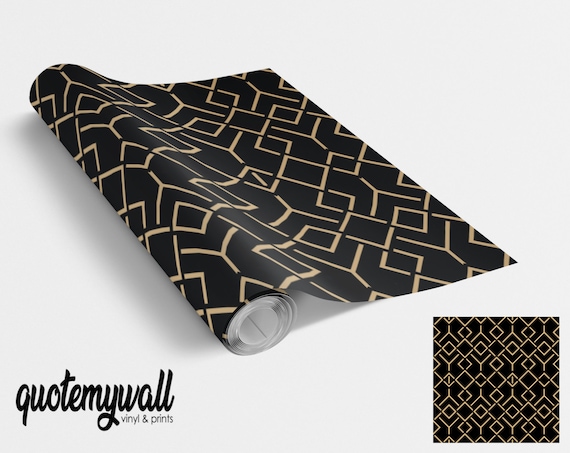The photograph showcases a product advertisement for a designer wallpaper roll on a white background. Positioned diagonally and partly unrolled by about eight to nine inches, the roll features an intricate black and gold pattern composed of diamonds and Y-shaped elements. The unrolled section provides a clear view of the design. In the bottom right corner, a square sample displays the entire pattern in a flat layout, emphasizing its abstract and geometric nature with sharp lines and 90-degree angles. The bottom left corner includes text reading "quote my wall vinyl and prints," identifying the brand. The image skillfully combines elements to give a comprehensive visual understanding of the wallpaper's appearance and design intricacy.